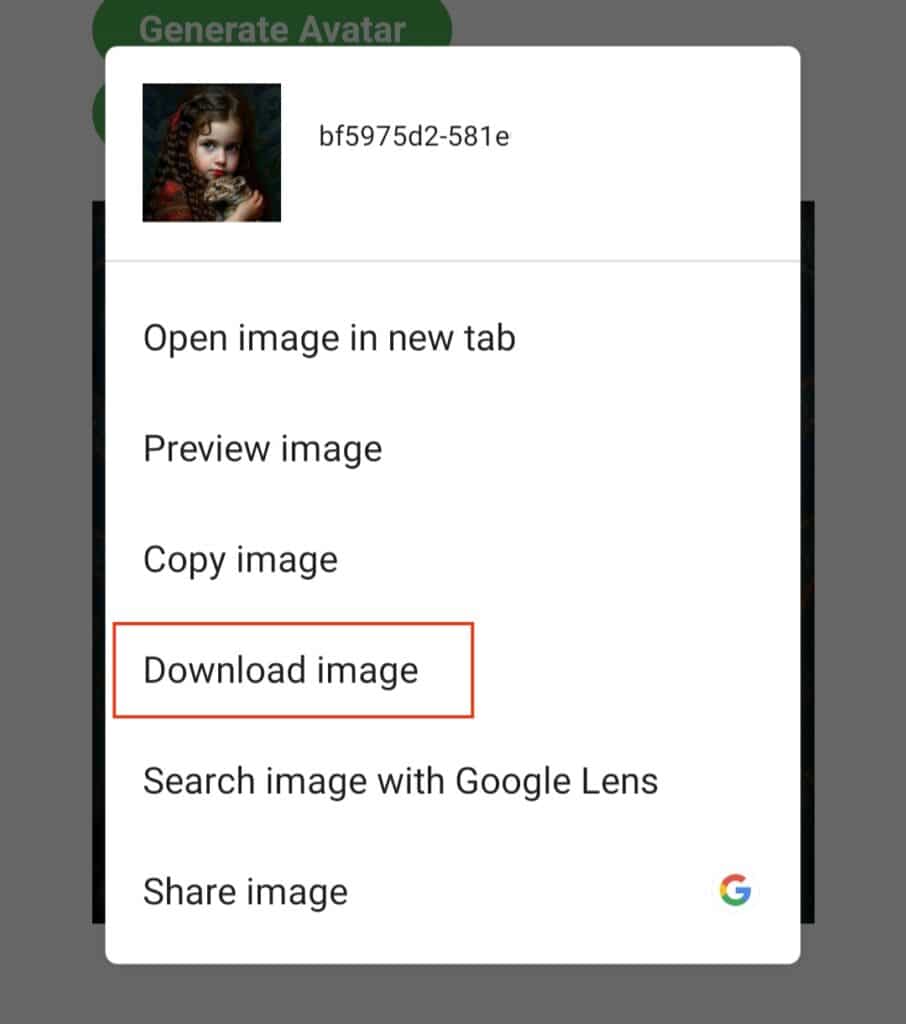The image is a screenshot of a website with a white pop-up overlay. The pop-up has a gray tint and contains the text "Generate Avatar Below." In the top left corner, there is a small photo of a little girl holding a ferret. The girl has white skin, brown curly hair, and is wearing a red dress with a matching red bow in her hair. She has red lips. Next to the photo, a code "BF5975D2-581E" is displayed. Below this, there is a list of actions separated by lines: "Open image in new tab," "Preview image," "Copy image," "Download image," "Search image with Google Lens," and "Share image." The "Download image" option is highlighted with a red outline shaped like a combination of a triangle and a rectangle. At the bottom right corner of the pop-up, there is a small icon of the Google "G." The webpage behind the pop-up is mostly obscured, with visible colors including green, white, red, black, brown, pink, yellow, blue, and gray. The pop-up covers the majority of the screen and is taller vertically than it is wide.